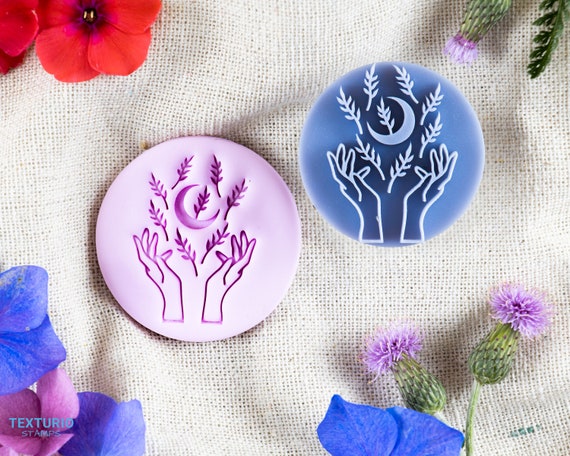This is a detailed photograph showcasing two perfectly round ceramic pieces, potentially buttons or rubber stamps, set against a white cloth background that resembles canvas. Surrounding these items are flower petals in various colors: red petals in the upper left, blue and purple petals in the bottom left, and a blue petal along with green flower buds topped with purple in the bottom right. The ceramic piece on the left has a light pink background and features a raised image in purple of two hands, depicted from the wrist up and forming an antler shape, gesturing upwards. Above the hands are small wheat-like branches and a crescent moon. The piece to the right, set slightly higher, mirrors the same design but with a light blue background and white elements. Both items are centrally placed in a diagonal alignment, adding symmetry to the composition.